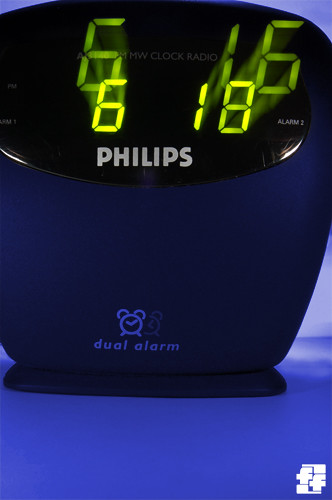The image depicts a close-up photograph of a digital alarm clock, potentially designed for promotional use. The clock itself is labeled "Philips Dual Alarm" and features a small icon in the bottom right corner, possibly bearing the letters "FF." The alarm clock is designed with a sloping plastic body that appears to be dark blue, though it might also be perceived as dark purple. It has a black plastic digital display showcasing greenish-yellow numbers, which are slightly blurred to give the impression of being projected onto a wall or surface. The time displayed is 6:18. In addition to the time, the display includes text that reads "MW Clock Radio," "FM 1," and "Alarm 2." The clock also features a miniature image of a classic alarm clock with two bells on top.